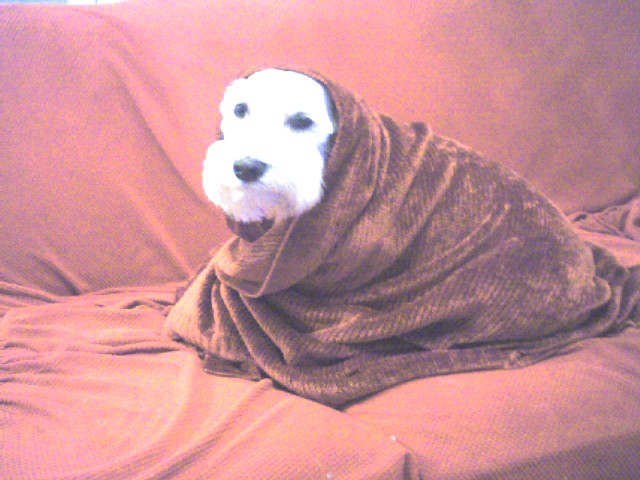This photograph, though slightly out of focus and of lower quality, captures a poignant moment of a small West Highland White Terrier, or Westie, wrapped snugly in a cozy, brownish-gold, corduroy-like blanket. The dog's white, shaggy fur, particularly evident around its bearded chin, stands out against the blanket and hints at its characteristic charm. The blanket is pulled up to cover its ears, enveloping the dog entirely except for its expressive face. The Westie's dark, black eyes and nose give it a slightly melancholic expression as it gazes slightly off-center towards the front of the picture. The setting appears to be an older couch which is itself draped in an orangish-red wrinkled cover, contributing to the overall tenderness of the scene. The image's vintage quality, without any visible people or text, adds to the nostalgic and intimate atmosphere.